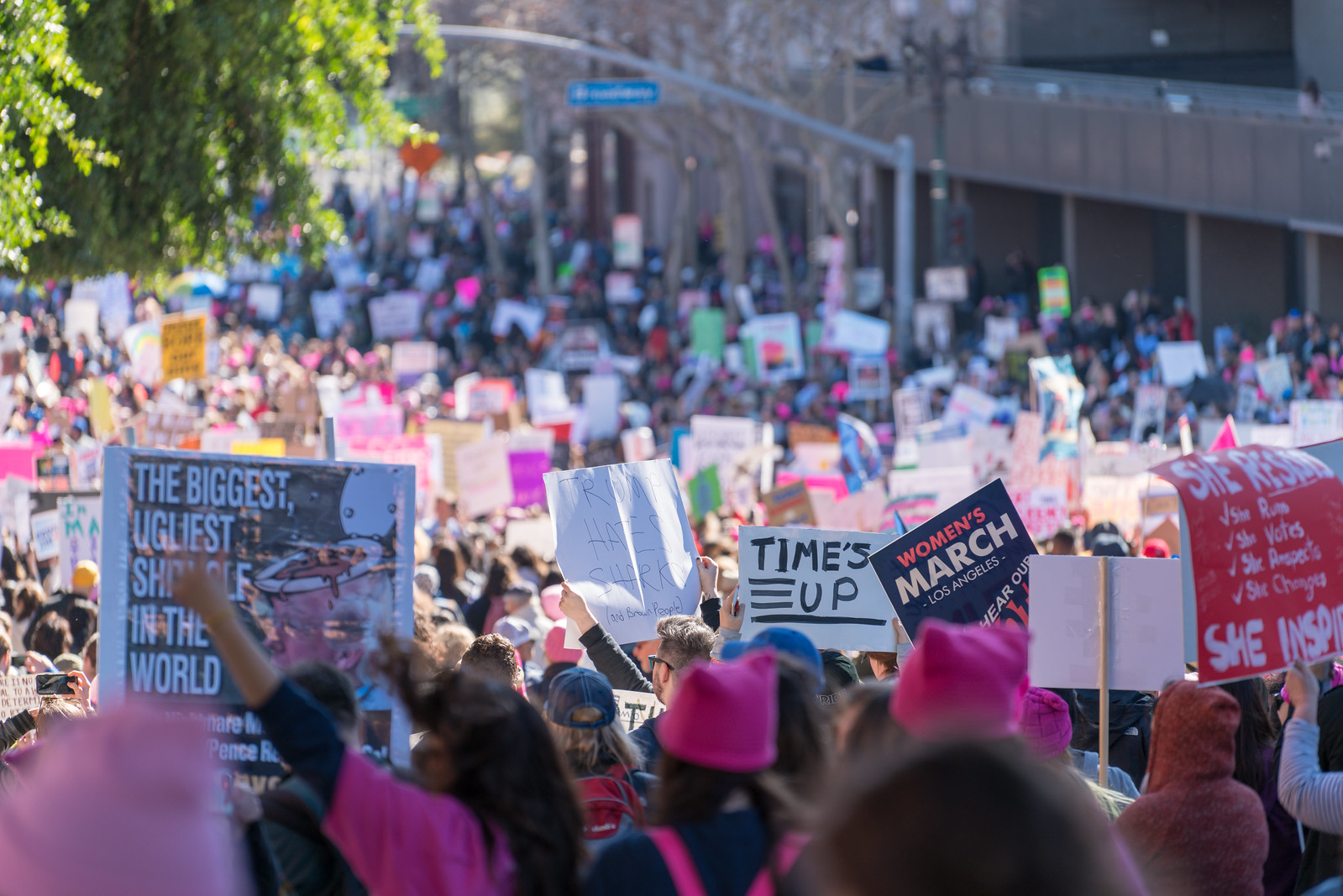The photograph captures a densely-packed street filled with protesters participating in a women's march, advocating for women's rights. The crowd, predominantly wearing pink knit hats, all face away from the camera, holding various signs. Prominently in the center, one sign reads "Time's Up," while another to the right announces "Women's March Los Angeles." A notable sign in the lower left corner declares "The Biggest, Ugliest Shithole in the World," accompanied by an image of a toilet. Additional signs slightly obscured in the crowd include phrases like "Trump hates sharks" and "She resides, she votes, she changes." The upper left corner of the image shows trees with sunlight glaring off the leaves, while the upper right corner features a faint building. A blue street sign on a pole is visible but unreadable due to blurriness. The overwhelming presence of pink hats and diverse signs highlights the spirited and large-scale nature of the protest.